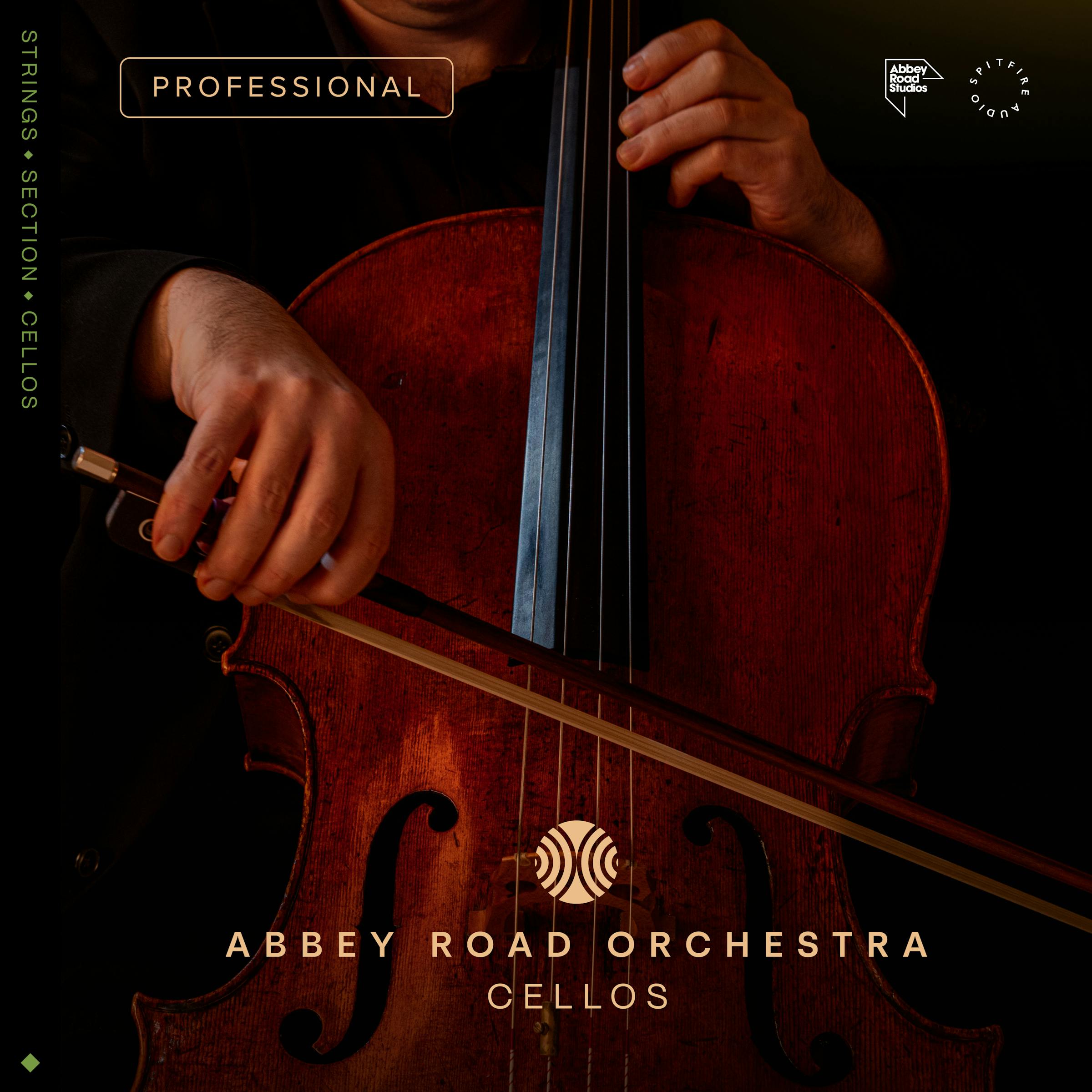The image is a detailed photograph of a cello being played, capturing the hands, the bow, and the upper three-quarters of the instrument, with the top portion and the tuning pegs out of view. The player’s lower chin is slightly visible, accentuated by a dark background that isolates the subject. The cello itself is a rich, dark brown, and the player's fingers are positioned to suggest they are pressing on the strings.

On the left side of the image, the text is arranged vertically and reads “strings · section · cellos.” In the top left corner, the word “professional” is displayed, while the iconic Abbey Road Studios logo is situated in the upper right corner, accompanied by a circular emblem with concentric semi-circles. At the bottom, bold text announces “Abbey Road Orchestra,” with “cellos” just beneath it. This combination of elements suggests the image may serve as an advertisement, possibly resembling an album cover or promotional material for a professional cello section recording at Abbey Road Studios.